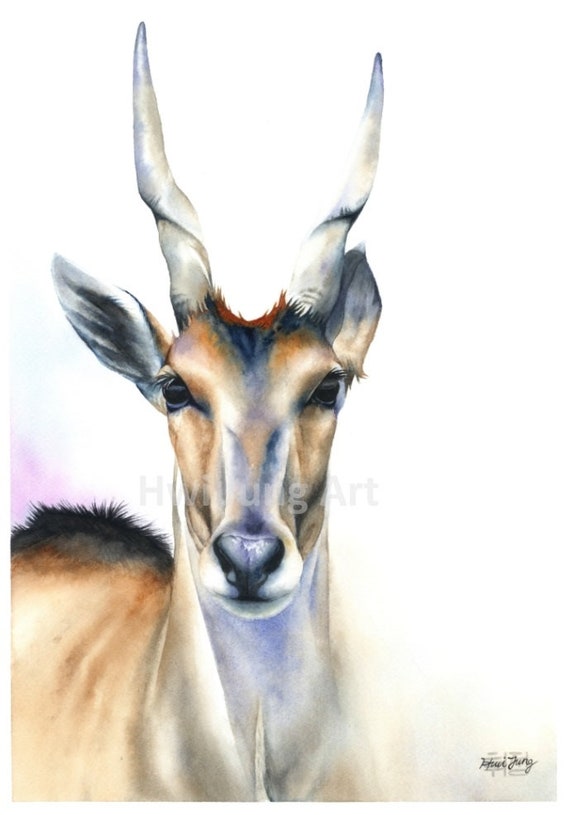The image is a captivating watercolor painting of an antelope, featuring the animal looking directly at the viewer with penetrating black eyes. The artwork is primarily focused on the antelope's head, which dominates the center of the composition. The head is adorned with distinctive long white horns that twist slightly, reminiscent of mythical dragon horns, adding a fantastical element to the piece. The facial details are intricately depicted: a large black nose centered above a mouth surrounded by white fur, while the rest of the face transitions into shades of light brown and black, with subtle purple hues highlighting certain areas. The antelope's large ears, which are black and white on the insides, frame the head, adding to the realism of the painting.

The neck and a portion of the antelope's back are visible, primarily on the left side of the image. The fur on the back is light brown with a distinctive black patch at the top. The use of watercolors gives the painting a wispy and ethereal quality, emphasizing the fluidity and grace of the animal. The sparse white background further accentuates the antelope as the focal point of the artwork.

Across the middle of the page, a faint watermark reads "HWI...UNG art," partially obscuring the details, and a small black signature accompanied by a stamp is located at the bottom right corner. The combination of these elements results in a mesmerizing and detailed portrayal of the antelope, capturing its essence with a blend of realism and artistic creativity.